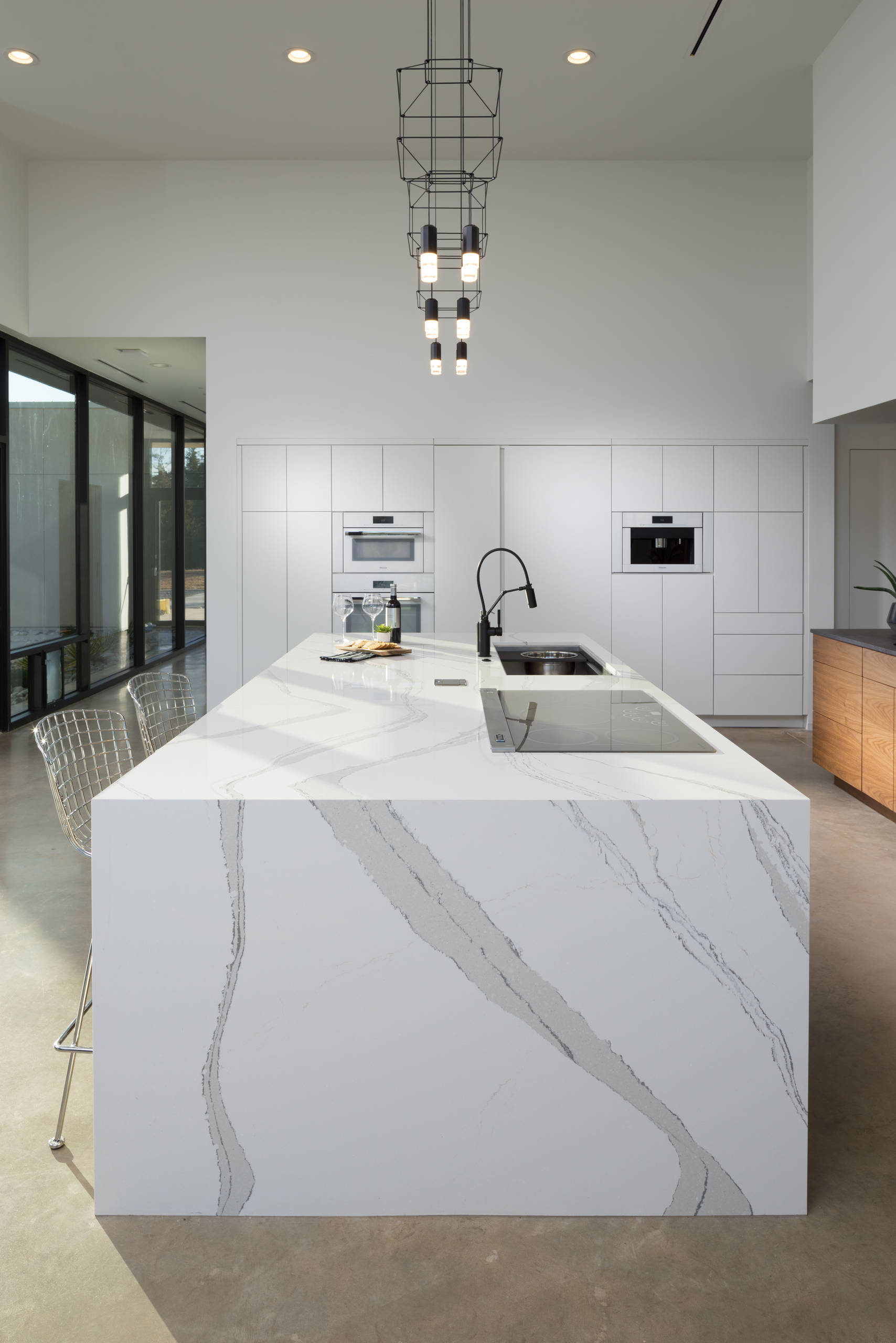This interior photograph captures a high-ceilinged, ultra-modern kitchen space characterized by its minimalist design and sleek aesthetics. The image is vertically oriented and prominently features a central marble kitchen island with a light and dark gray marbled surface. The island is equipped with a black rectangular sink that has a matching high-arched black faucet, and an adjacent cutting board area. Various objects, such as a wine bottle, two wine glasses, a bottle of oil, and a plate filled with bread, are neatly arranged on the island. In front of the island are two modern silver metal chairs.

The kitchen has a cohesive white color scheme, with white-tiled walls and integrated appliances, including a microwave and stove, that seamlessly blend into the walls. The right side of the image shows a refrigerator that continues this sleek, built-in look. Traditional wooden cabinets with clear countertops are seen in the background, adding a touch of classic elegance amidst the modern furnishings. The floor of the kitchen is paved with beige tiles, contrasting subtly with the purity of the white walls.

Above the island, the lighting is provided by modern, square chandeliers and a black wrought iron chandelier with six small white bulbs, hanging from a ceiling featuring recessed lights. A hallway on the left side of the image, leading to another room with ceiling-to-floor glass windows encased in white frames, suggests an open and airy layout. This immaculate kitchen, with its clean lines and integrated design elements, epitomizes a contemporary minimalist aesthetic.